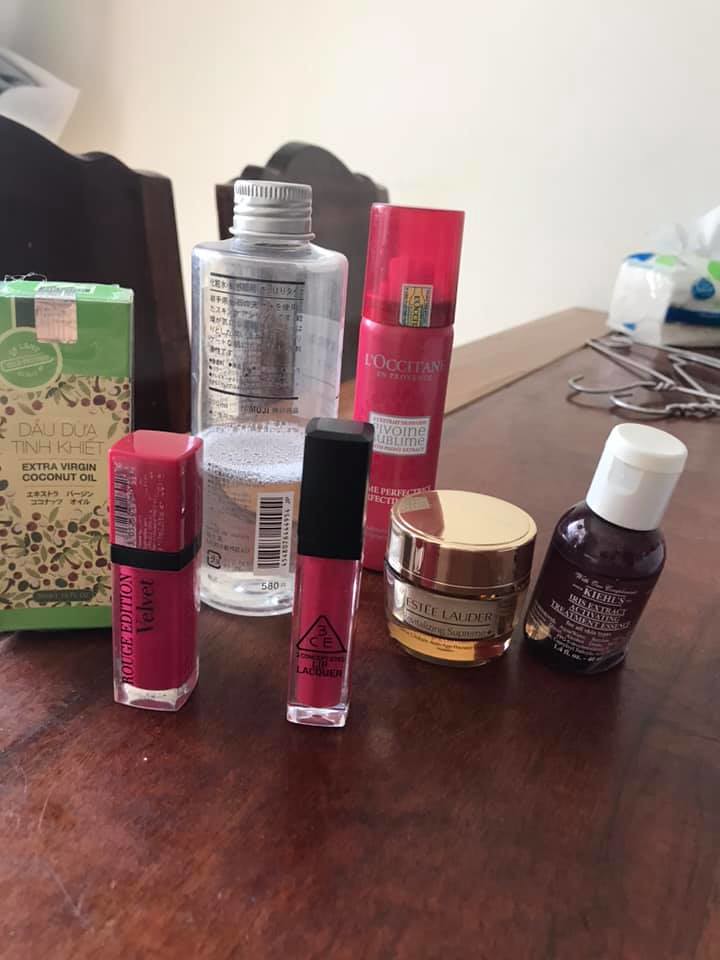The image features a neatly arranged collection of makeup products on a wooden tabletop. In the forefront, there is a prominent lipstick. Next to it on the right is another lipstick-type container with a square top. Further right, there is a container with a gold top that reads "Jessie Lanier." To the right of the gold-topped container, a small bottle with a white cap is visible. To the extreme left is a box labeled "Extra Virgin Coconut Oil." Centrally positioned and behind the lipstick is a container with a silver cap, displaying information on its back. To the right of this silver-capped container, there is a bottle of hairspray. The entire setup is on a wooden desk, with chairs visible in the background. Hangers are laid out to the right side, adjacent to a container of makeup wipes in the corner. The makeup collection includes six containers, three of which are pink.